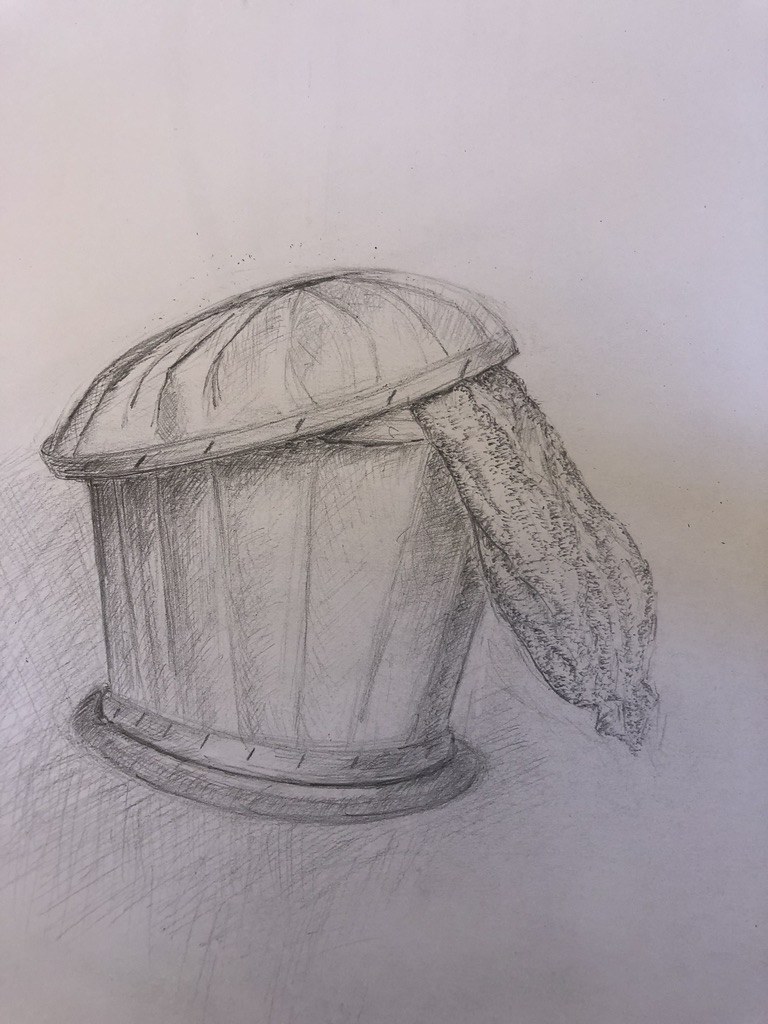This detailed black-and-white illustration, possibly created with pencil or charcoal, portrays a round container that resembles a garbage can, occupying three-quarters of a faint grayish-pink-tinted white paper. The container features vertical lines running along its entire body, enhancing its cylindrical shape, and rests on a darker base that gives it depth. The lid, which is dome-shaped and adorned with matching vertical lines, is slightly ajar and tilts to the left. Emerging from the open top is a long, narrow, and pointy object, reminiscent of a garbage bag, with pronounced shading indicating its weight and texture. The bag appears to take on the shape of a human body, adding an element of intrigue. Subtle lines and shadows are skillfully employed around the container and the hanging bag, creating a shiny effect and further emphasizing the detailed craftsmanship of the illustration. Surrounding the lower part of the container, the background is slightly shaded, grounding the object within the scene.